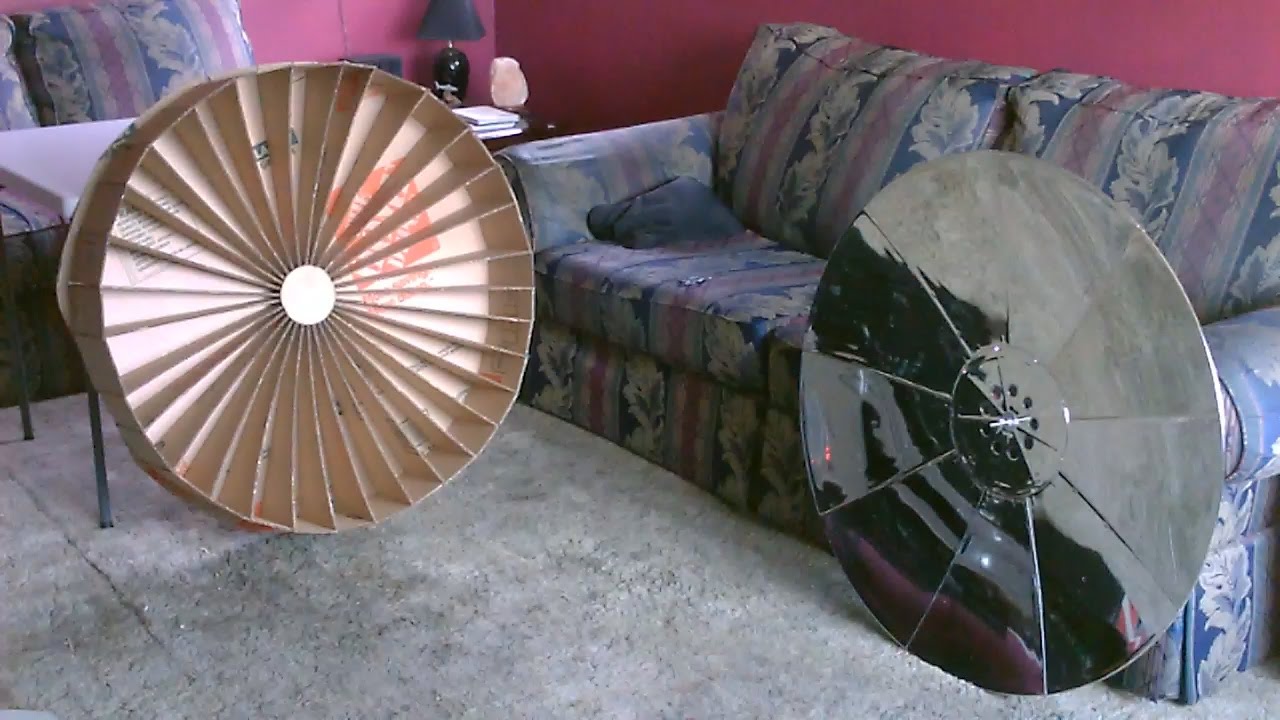In this detailed indoor image, we're looking at a rather cluttered and dusty living room, viewed in landscape orientation. The focal point is the pair of matching, vintage couches situated along the back walls, which converge in a corner. These old, stained couches feature a pattern of vertical stripes in red, blue, and white, combined with a floral design, evoking a dated, art deco ambiance. Adjacent to where the couches meet is a slightly obscured table adorned with a black lamp, possibly with a blue shade, accompanied by several white books or notepads.

The living room's walls are a deep, purplish-red hue, adding to the overall saturated and nostalgic atmosphere. On the left side of the room, beside the couch, is a unique gold steel drum with approximately 30 fan blades encircling its bronzy circumference. On the right, a silver metallic reflector-type disc leans against the couch, mirroring a similar wheel-like contraption fashioned from cardboard and a piece of Home Depot cardboard, creating an impression of makeshift, man-made objects.

The carpet, a light gray, is notably grimy and covered with dust or dirt, especially piled up in the center. Adding to the room's eclectic detailing is a small white table with black legs housing a constructed wheel-type object facing the camera. This combination of elements — the worn furniture, the peculiar objects, and the vivid wall color — collectively paints a picture of an interior space rich with character, albeit in dire need of a thorough cleaning.